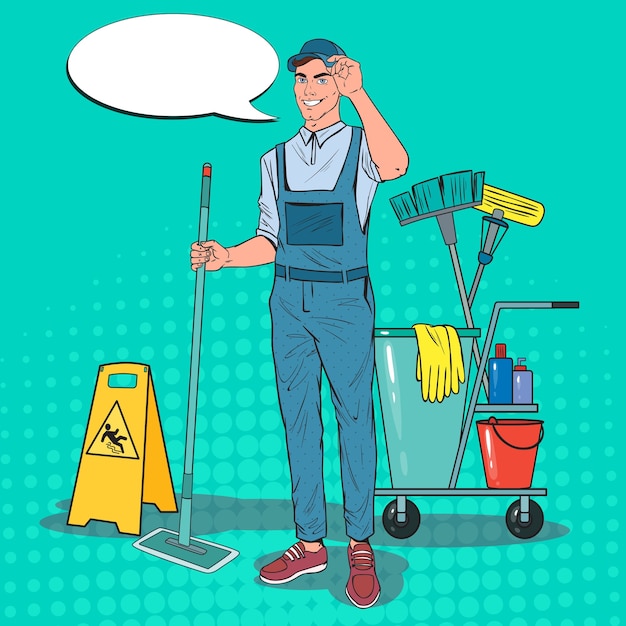The illustration features a cartoon janitor on a teal blue background with lighter blue dots rising halfway from the bottom. The janitor is wearing dark blue jean overalls and a light blue button-collared shirt. He is sporting a blue baseball cap, which he is holding with his left hand in a gesture as if to greet or tip his hat, smiling warmly. His right hand holds a Swiffer Sweeper broom, which has a turquoise-type green interior and a black outline.

The janitor stands in front of a janitor cart, which is detailed with various cleaning supplies: a blue can, yellow gloves, a blue and yellow broom, a blue bottle, a purple bottle, and a red bucket with black wheels. Additionally, a caution sign showing a silhouette of a person slipping is positioned to the left, indicating "Slippery When Wet." The janitor is wearing burgundy-colored tennis shoes with white laces, and there's a white speech bubble above him to the left corner, although it is blank.